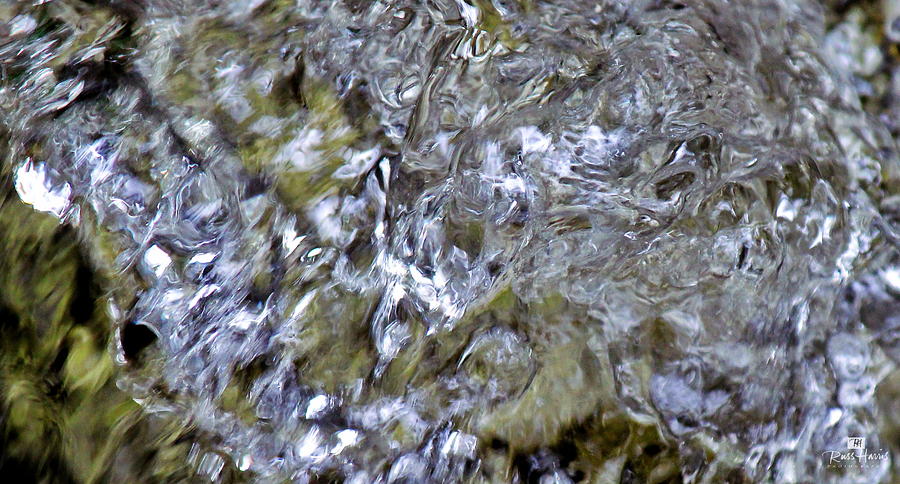The rectangular image showcases a turbulent and abstract close-up of fluid, possibly water, ice, or plastic, flowing in various directions with swirls of white, silver, brown, yellow, and black creating a complex pattern reminiscent of the texture you might find on an animal or statue. The chaos and motion make it difficult to discern any specific objects within the composition. In the blurred background, a hint of green can be seen, suggesting a possible plant. Adding to the artistic confusion is a small, distinct logo located in the bottom right corner, featuring the initials "R.H." above the name "Russ Harris" in a white script font, with "photography" written below in a different style, subtly identifying the creator amidst the swirling chaos.